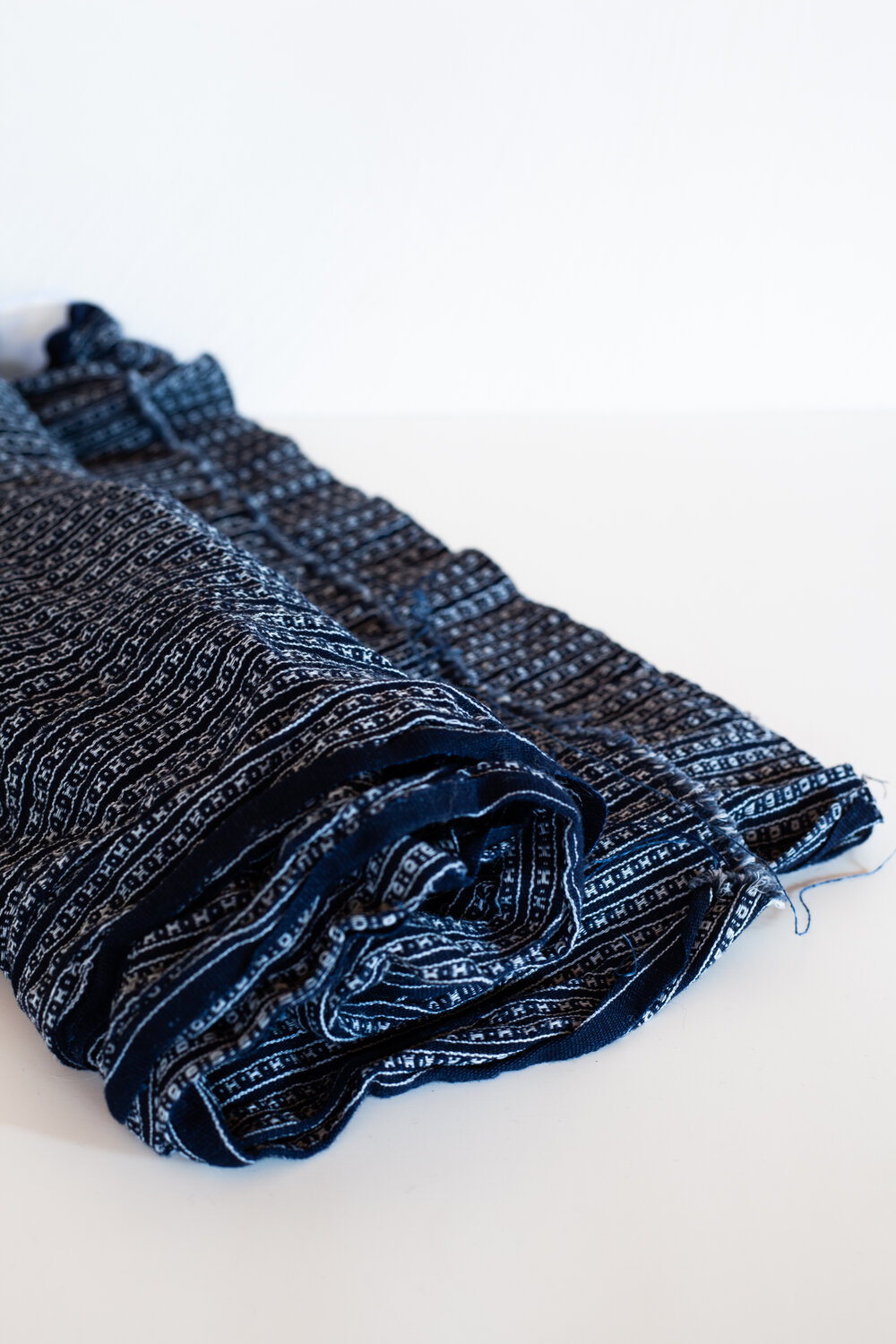The image features a piece of dark navy blue cloth adorned with a distinct white pattern, set against an entirely white background. The cloth, which appears to be either a placemat or a scarf, is characterized by a series of horizontal stripes alternating between solid blue and thin white stripes. Within the white stripes, there is a repeated H-shaped design. The cloth is rolled up, starting from the left and spiraling towards the right, partially unrolled to reveal its intricate pattern and frayed edges. The fabric is laid out in a manner that it remains focused in the foreground, with the background subtly fading out of focus.